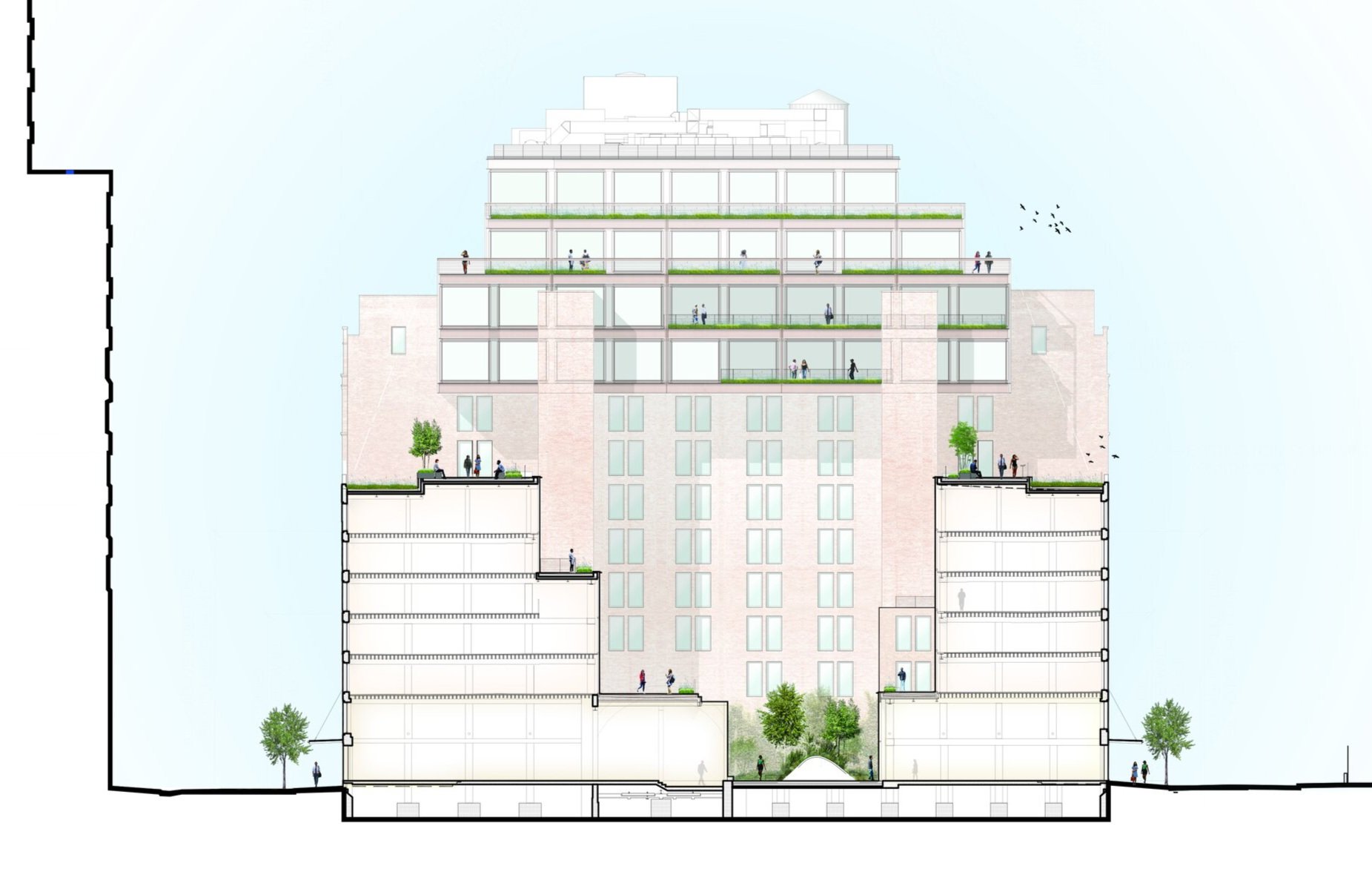The image is a detailed sketch drawing of a tall, multi-level building that appears to be either an apartment complex or a large hotel. The building is depicted in white and light pink, with many windows and balconies. As the building ascends, it narrows and features large floor-to-ceiling windows.

Two large trees flank either side of the building, and smaller trees are scattered around the base, with some areas of green grass visible. People can be seen standing and walking on the upper balconies and terraces, which have guardrail fences and appear to be the most expensive units. The terraces also have sections where grass is growing.

The background of the sketch has a light blue hue, outlined with a black zigzag pattern, and there appear to be birds flying on the right side of the building. Along the bottom left side, there is a man dressed in white and black standing next to a green tree. There are also indications of steps leading up to the building and smaller underground apartments with small windows.

To the right, there is another tree with two people standing nearby, dressed in dark clothing. The entire composition includes a variety of people in different locations, adding a lively atmosphere to the scene.